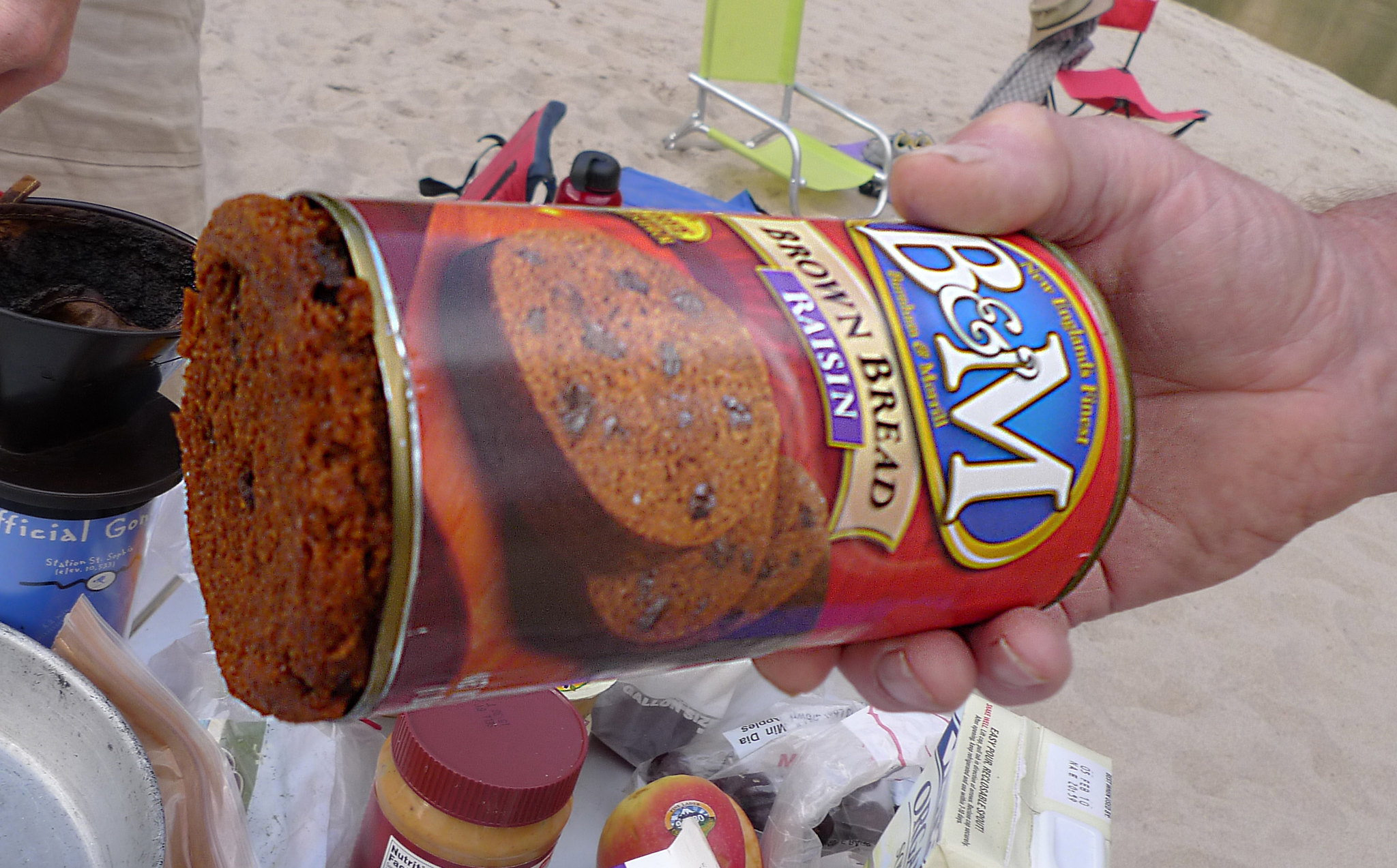In this brightly lit beach scene, a man’s hand prominently extends from the right side of the frame, holding a quirky can of B&M Raisin Brown Bread. The can, vibrantly labeled in red with the brand name "B&M" in bold white lettering encircled by blue, grabs immediate attention. Its bottom has been removed, allowing the dense bread to peek out. The backdrop is a sun-drenched stretch of light brown sand, reinforcing the beachside ambiance. At the top of the image, two beach chairs in festive green and red fabrics hint at a lazy, relaxed atmosphere. In the lower part of the photo, the scene is completed with a scattered setup of picnic essentials – a jar of peanut butter, a plump fruit that appears to be either an apple or a peach, and a handful of napkins, suggesting preparations for a casual beachside snack or picnic.